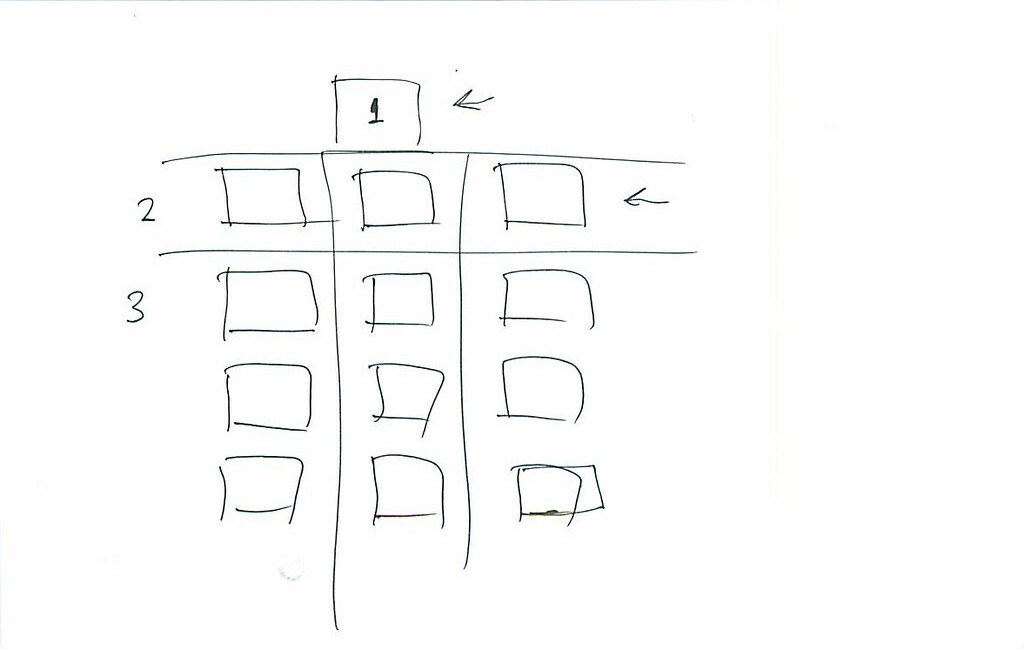In the image, a person is drawing on a piece of paper. The paper is divided into three rows, with only one horizontal line drawn across the top. The top row features a partially enclosed square box with the number "1" inside it on the left side. Adjacent to this box, on the right side, is an arrow pointing left towards the box.

In the second row, there are three roughly sketched square boxes aligned next to each other. Similar to the first row, an arrow on the right side points towards the boxes.

The third row has the number "3" on the left side, followed by nine poorly drawn square boxes, arranged in a 3x3 grid. Once again, an arrow on the right side points towards these boxes.

Overall, the drawing appears unrefined, with inconsistent line lengths and no use of any measuring tools. The numbers and boxes are drawn freehand, without precise alignment. Additionally, in the bottom right corner, there is an erratically drawn figure that resembles the number "7," but its clarity is compromised by the hasty drawing style.